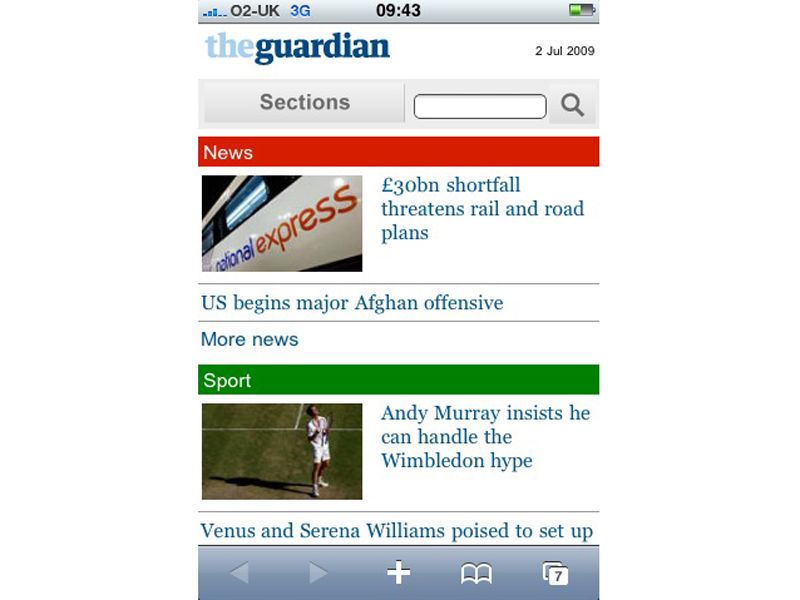This is a mobile phone screenshot capturing a moment from The Guardian app on July 2, 2009. At the top, a grey status bar displays typical phone information: on the left, a mobile signal icon shows 3 out of 5 bars next to the text "O2-UK" in black font, a "3G" indicator in blue font, and the current time "09:43" in black font. On the right side of the bar, a half-filled battery icon is present.

The main content of the screenshot features a white background with "The Guardian" in blue font and the date "2 July 2009" in black font above a grey navigation bar. This bar includes a "sections" button depicted in darker grey font, and an empty white search field containing a black magnifying glass icon on its right.

Below this navigation bar, a red rectangle with white font reads "News." Positioned beneath it is an image of a National Express bus, followed by the headline, "£30 billion shortfall threatens rail and road plans." Another news headline, "US begins major Afghan offensive," is situated below the first, and under it, a clickable "More News" link is available.

Further down, a green rectangle with white font denotes the "Sport" section. Below this section title is an image of a man clad in a tennis uniform, holding a racket and looking skyward.